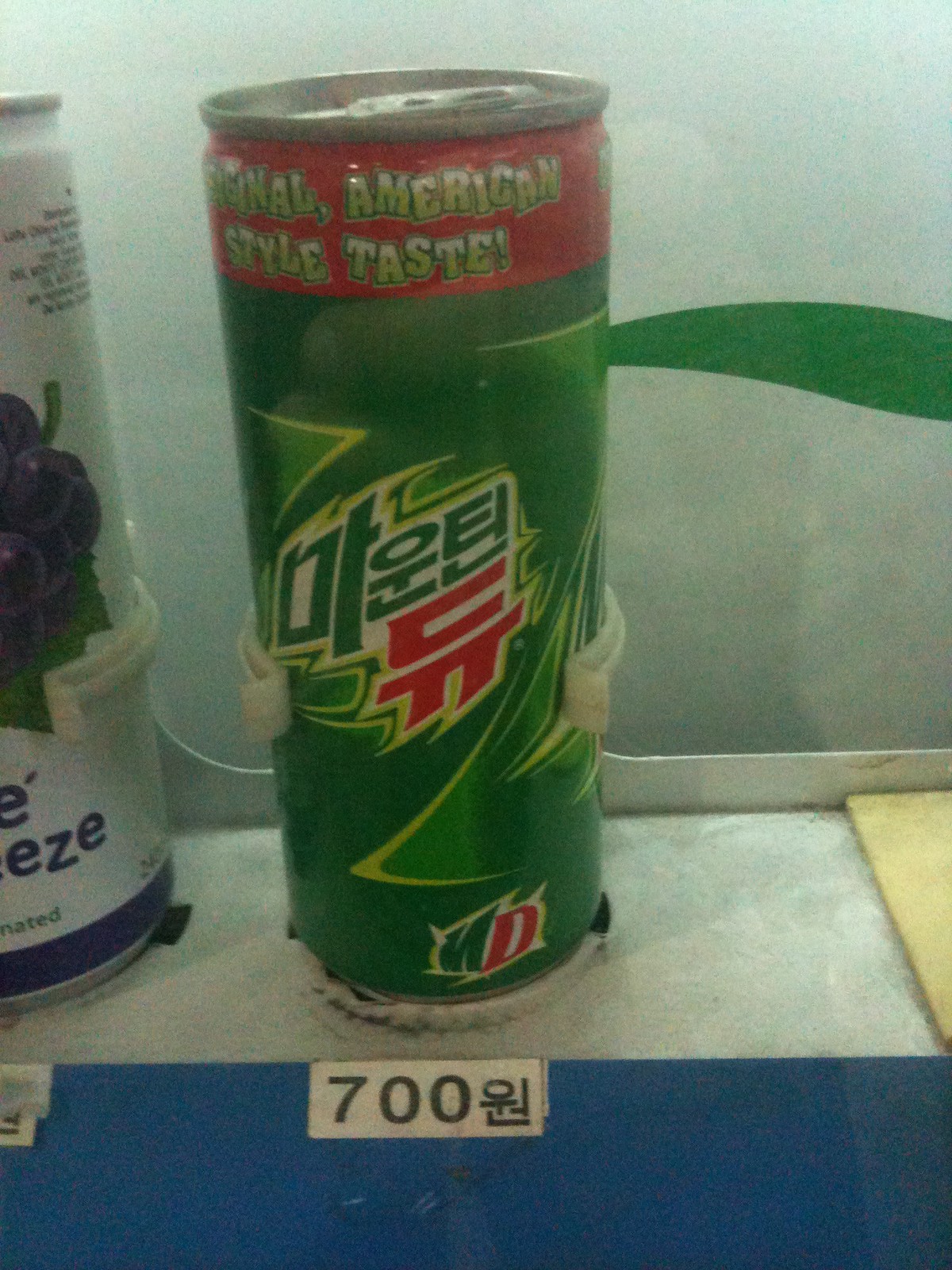The image showcases two cans positioned on a white platform. The can in the center is fully visible, while the one on the left is partially obscured. Behind the cans, the background is predominantly white, with a green stripe running vertically along the right side. The foreground features a blue platform with a label displaying the number "700" alongside a Korean character, all written in black text. The central can is prominently displayed against a red background adorned with the words "SIGNAL, AMERICAN, STYLE, TASTE,!" in bold lettering.